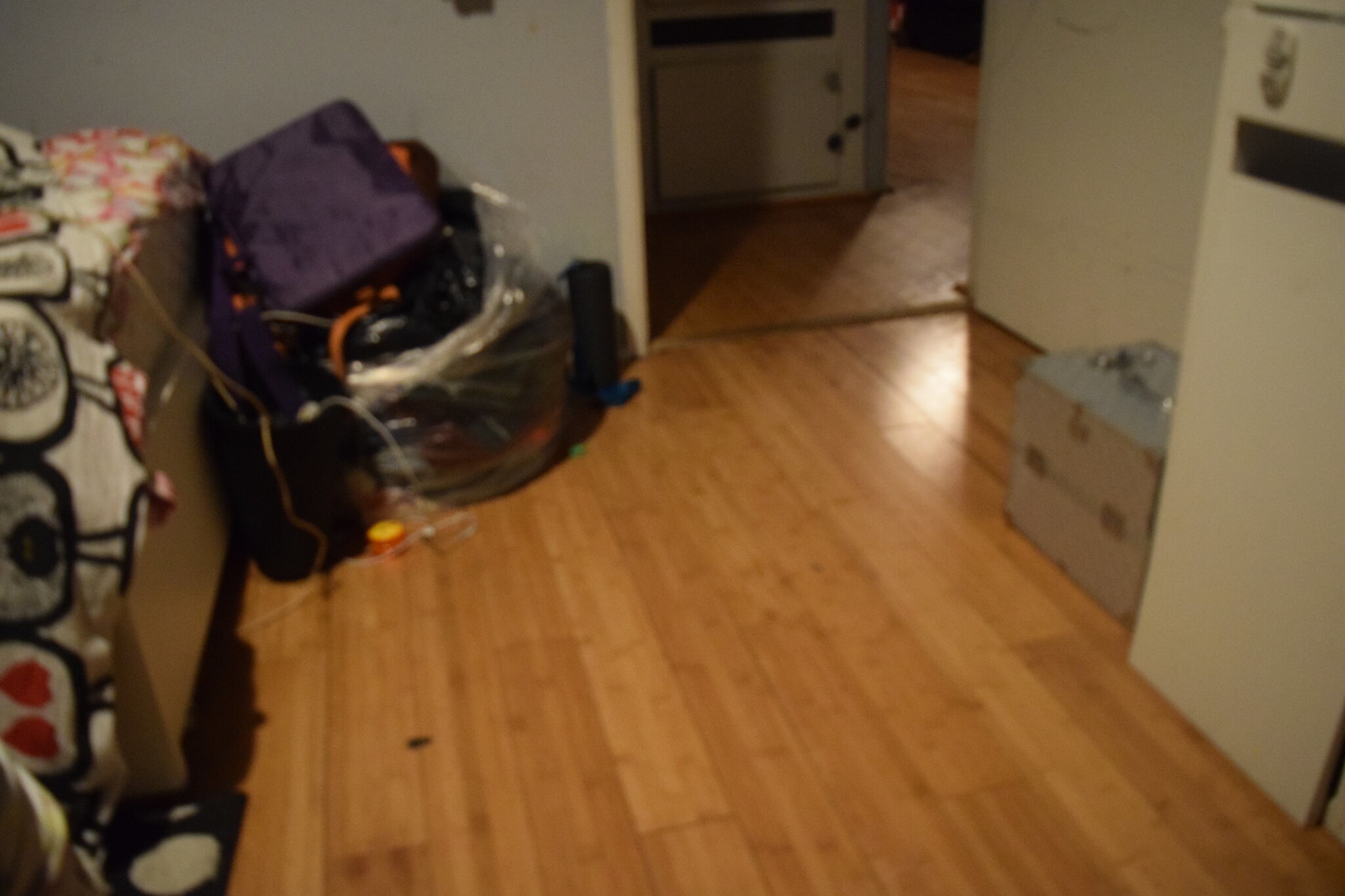This photograph captures the slightly blurred interior of a cluttered bedroom with laminate or hardwood floors. To the left, the edge of a bed is visible, adorned with a patterned duvet cover featuring a whitish background and large black circles interspersed with red or black dots. Centered in the image is a doorway leading to a hallway, featuring a white door equipped with a rectangular doggie door. In front of the bed, a haphazard pile of items includes bags and containers, notably a clear plastic bag filled with fabrics and topped with a purple suitcase or box. On the right side, a white-painted cabinet stands next to a closed silver trunk with whitish silver buckles and a carry handle, resembling a camera or electronic equipment case. The room has a light brown wood floor that extends through the visible area. The overall scene suggests a lived-in, somewhat disorganized space.